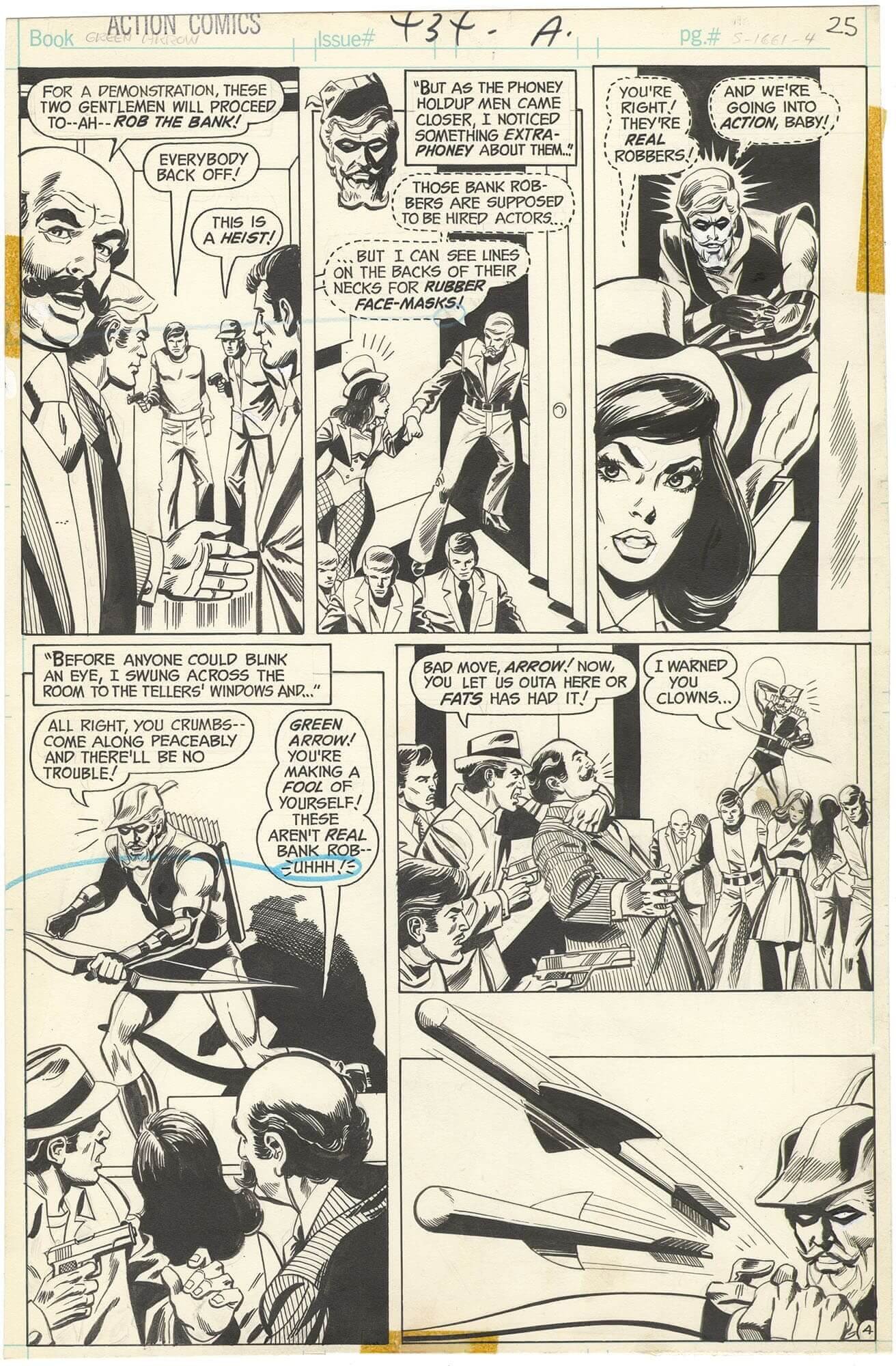The image displays a page from a black and white cartoon or graphic novel, likely a Green Arrow comic, printed on slightly yellowed paper with rough edges, possibly indicating it was taped into an album. At the top left, text labels read “book” followed by a horizontal line; then “issue” with a hash symbol; continuing with “P” in capitals, “g” in small, a dot, and another hash symbol. Next to “book,” green text accompanies black, all-caps text that says “Action Comics,” slightly cut off at the top. Near “issue,” handwritten text in black ink reads “434-A,” and beside the “page” label, faded numbers are almost illegible, except for a clear “25” to the right.

The comic strip features five panels arranged in a vertical and horizontal layout. The first panel introduces a group of people in a bank, with speech bubbles indicating a demonstration as two men stage a heist: “Everybody back off, this is a heist.” The second panel reveals a character, possibly Green Arrow, recognizing the robbers as imposters wearing rubber masks: “But as the phony hold-up men came closer, I noticed lines on their necks.” The third panel confirms the real robbery, showing Green Arrow preparing for action: “We’re going into action, baby.” The fourth panel, on the bottom left, depicts Green Arrow swinging towards the tellers, confronting the robbers: “Come along peaceably and there’ll be no trouble.” The next panel to the right shows one of the robbers threatening a hostage: “Now you gotta let us out of here or fats has had it.” In the final panel, Green Arrow retaliates, drawing arrows from his quiver: “I warned you clowns,” as he begins his counterattack.